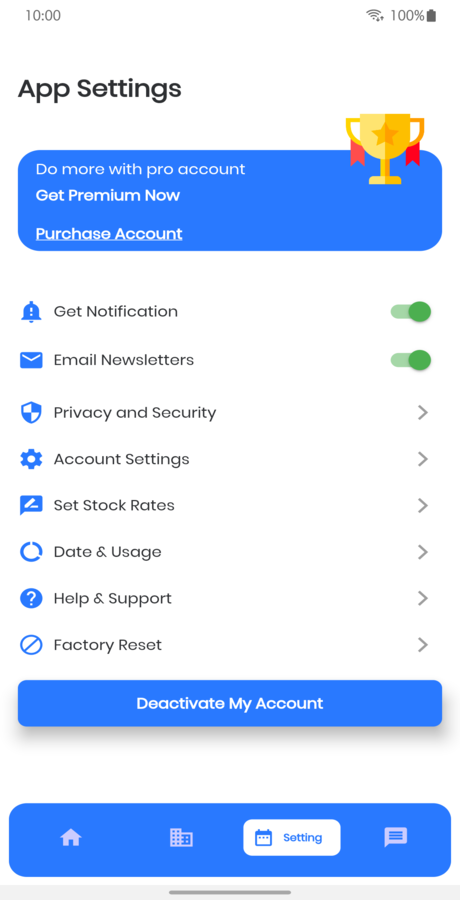This image shows a screenshot of a cell phone screen displaying the settings menu of an app. At the very top, the status bar indicates the time is 10:00 AM, and the battery is fully charged at 100%. Below the status bar on the left, the header "App Settings" is written in black text.

Directly beneath the header is a promotional banner with a blue background, urging users to upgrade to a premium account: "Do more with Pro account, get premium now." Adjacent to this message, on the top right corner of the banner, is an image of a gold trophy adorned with red ribbons on each side.

Following the promotional banner, there are nine setting categories listed in a vertical sequence:
1. Get Notification
2. Email Newsletters
3. Privacy and Security
4. Account Settings
5. Set Stock Rates
6. Data and Usage
7. Help and Support
8. Factory Reset

The first two categories, "Get Notification" and "Email Newsletters," feature green toggle switches to their right, both of which are in the 'on' position.

At the very bottom of the settings list, there is a blue button with white text that reads, "Deactivate my account." Further down, another blue background bar houses four icons:
- A house icon on the far left
- Two overlapping squares next to it
- A settings icon with a white background and blue text
- A message icon on the far right

Finally, at the absolute bottom, there is a small horizontal gray line centered at the bottom edge of the screen.